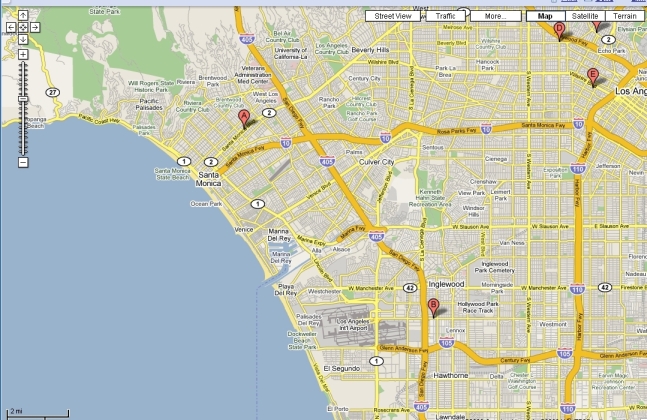This detailed map prominently features the coastal regions of California, highlighting the striking blue waters on the left side of the image. Notable areas such as Santa Monica and Beverly Hills are visible, along with key landmarks including the University of California, Los Angeles (UCLA), the Veterans Administration, and Marina del Rey. The map extends to encompass diverse neighborhoods like Inglewood, Echo Park, and Hancock Park within the sprawling cityscape of Los Angeles.

Moreover, the map interface is adorned with white squares containing black labels that provide options such as Street View, Traffic, More, Map, and Satellite views. Major highways are marked in bold yellow lines, with Interstate 10 running horizontally across the state and Interstate 405 descending vertically. Further south, Hawthorne is identified along with the intersections of Interstate 110 and Interstate 105, creating a comprehensive visualization of the region's complex transportation network.